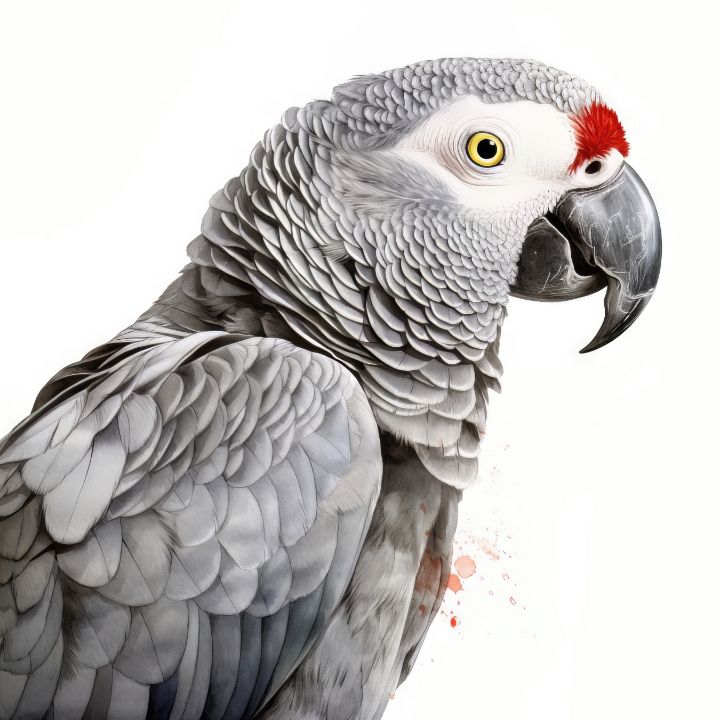Against a matte white background, the image showcases a detailed close-up of a gray parrot, cropped from the stomach up. The parrot's sharp, black beak—which shows some scratches and has nostril holes—is rounded and pointy, characteristic of tropical birds. Its eye is strikingly yellow with a black pupil, surrounded by bright white feathers. Above the beak is a deep red spot of feathers, giving the bird a distinctive and colorful facial feature. The parrot’s plumage varies in shades of gray, becoming slightly darker down the body, with lighter feathers adorning its abdomen. Notably, its folded wing and fluffy head feathers are visible. There is a peculiar detail on the bird's chest—red and white droplets that appear smudged, reminiscent of blood or a red juice stain, and seemingly unrelated to the parrot itself, suggesting an external spillage on the image.